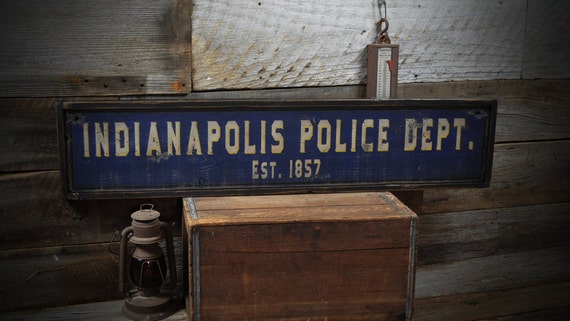The photograph depicts a vintage museum display featuring a variety of antique items set against a backdrop of distressed, horizontally-laid wooden planks. Central to the image is a small, closed wooden box, possibly reinforced with metal at the edges, which rests on what appears to be a concrete floor. Atop the box sits a rectangular sign framed in dark wood with a blue background. The sign reads "Indianapolis Police Department, established 1857" in tan lettering. To the left of the box is a tall, brown oil lantern or glass lantern with metal elements. In the background, behind the sign, is an old wooden wall composed of four long panels, and a vertical white object, possibly a gauge or thermometer, is faintly visible. The setting seems to be intentionally aged and weathered, evoking a sense of historical preservation.